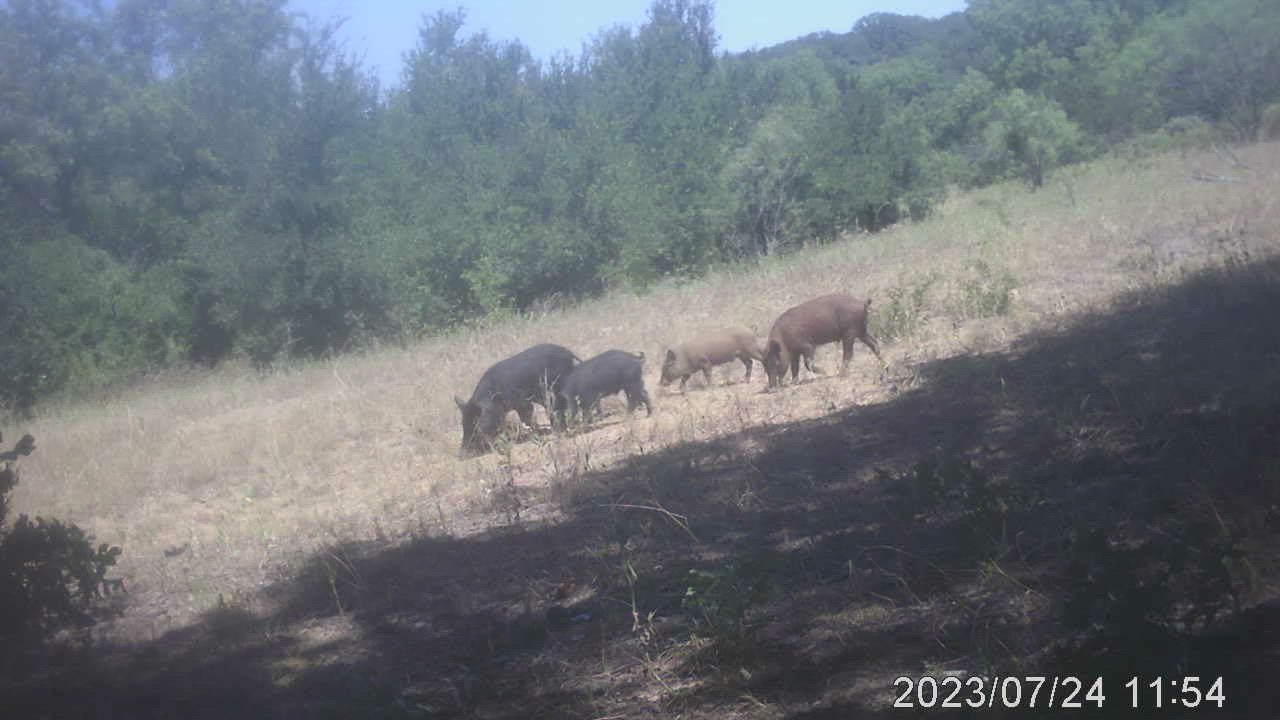This photograph, captured on a webcam with a timestamp reading "2023-07-24 1154," depicts a wildlife scene in a mid-summer, dry-looking field with some trees and a bright blue sky in the background. The image is horizontally cropped, very blurry, overexposed, and out of focus. The field's vegetation appears yellowed and sun-bleached, indicating the season's heat or drought conditions. The angle of the photograph shows a diagonal shadow from the bottom left towards the right middle section.

In the highlighted center strip of the image, four large animals resembling boars or warthogs are grazing. The lead animal, likely the largest of the group, is a dark brown or black color, possibly indicating it might be a male. Following it are three smaller animals of varying colors: another dark brown or black, one beige, and one brown. These animals are all focused with their heads down, likely foraging for food. The lack of visible enclosures suggests that these could be wild or feral animals. The background, though out of focus, shows a line of trees or tall bushes, adding depth and context to this outdoor wildlife scene.